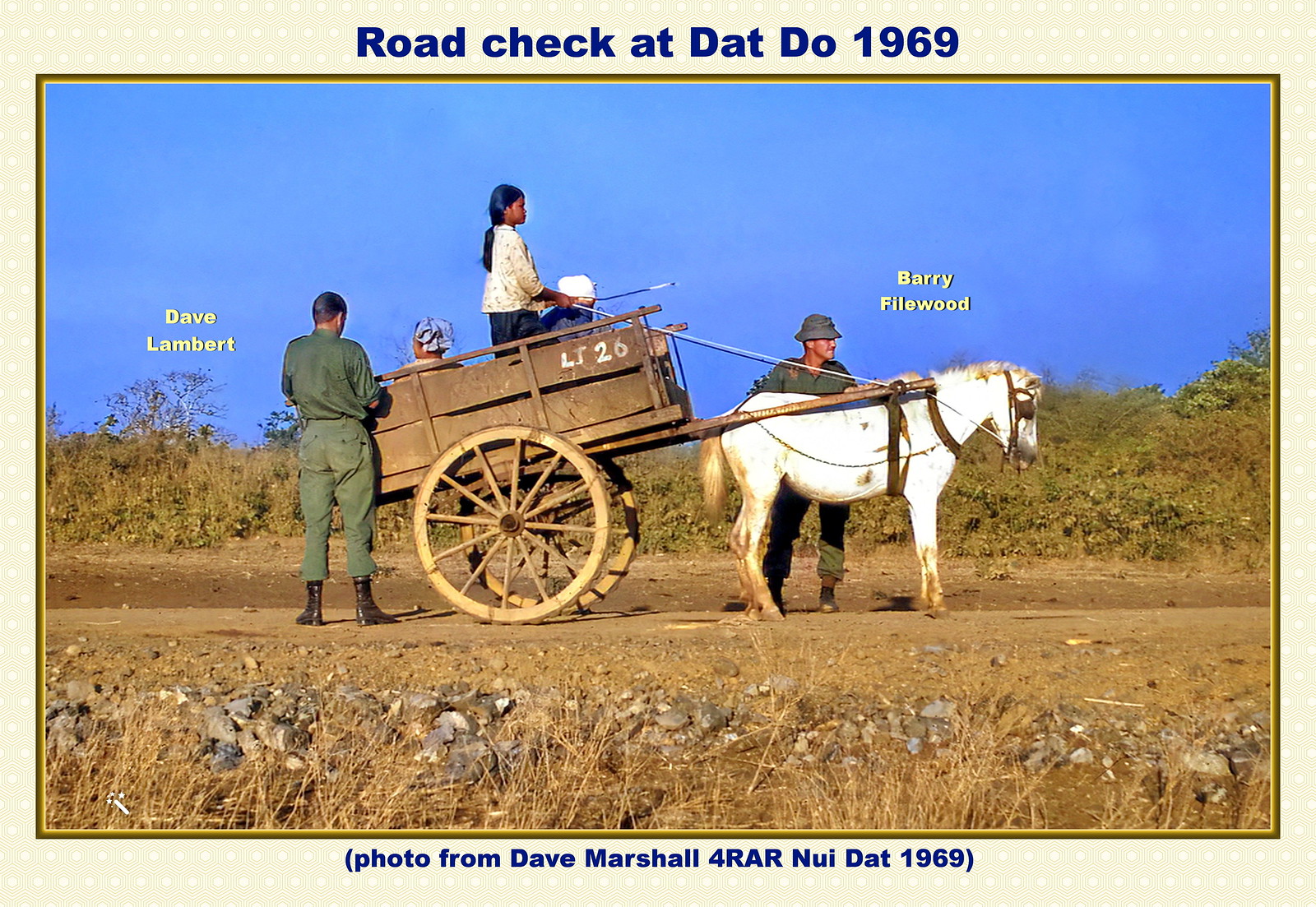In the photograph titled "Road Check at Bat Du 1969," we see a detailed scene captured during what seems to be a routine inspection on a dirt road. A white horse is positioned on the right side of the image, facing to the right, and is harnessed to a carriage with a wooden compartment atop two large wheels. On this wooden compartment, a young, dark-skinned girl with black hair pulled back into a ponytail is standing and facing left. Seated beside her on the left is another person.

To the far left of the wooden compartment, a man in uniform, identified as Dave Lambert, is facing away from the camera. Another uniformed man, labeled as Barry Filewood, stands closer to the horse on the right. The scene hints at a historical moment marked by the names and context: Barry Filewood and Dave Lambert are engaged in what appears to be a road check.

The road itself is a simple dirt path with minimal greenery, bordered by bushes and under a clear blue sky. The bottom of the image attributes the photograph to Dave Marshall and notes that it was taken for an entity referred to as ARA Newie in 1969.